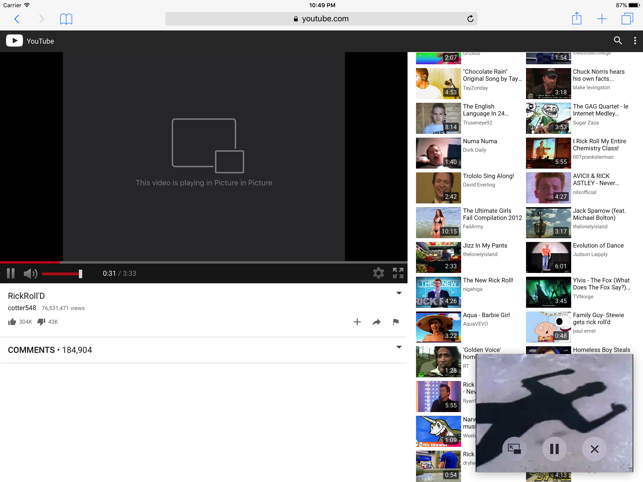Here is a detailed and cleaned-up caption for the image described:

---

The YouTube homepage displayed in the image features a URL of youtube.com. The main video screen, prominently in the center, has a black background with the text overlay reading "This video is playing picture-in-picture," despite no video currently playing. The video being highlighted is titled "Rick Rolled," which has amassed an impressive 76 million views. 

To the right of the main video screen, there are multiple thumbnails in a vertical column, each representing recommended videos. Each thumbnail displays an image alongside the video title and the uploader’s name. 

In the lower right-hand corner of the screen, there is a distinct screenshot of a man's shadow cast on concrete. The text accompanying various video thumbnails includes titles such as "Chocolate Rain" (Original Song by Tay), "The English Language in 24 Accents," "Nirma Nirma," and "Trololo Sing-Along."

---